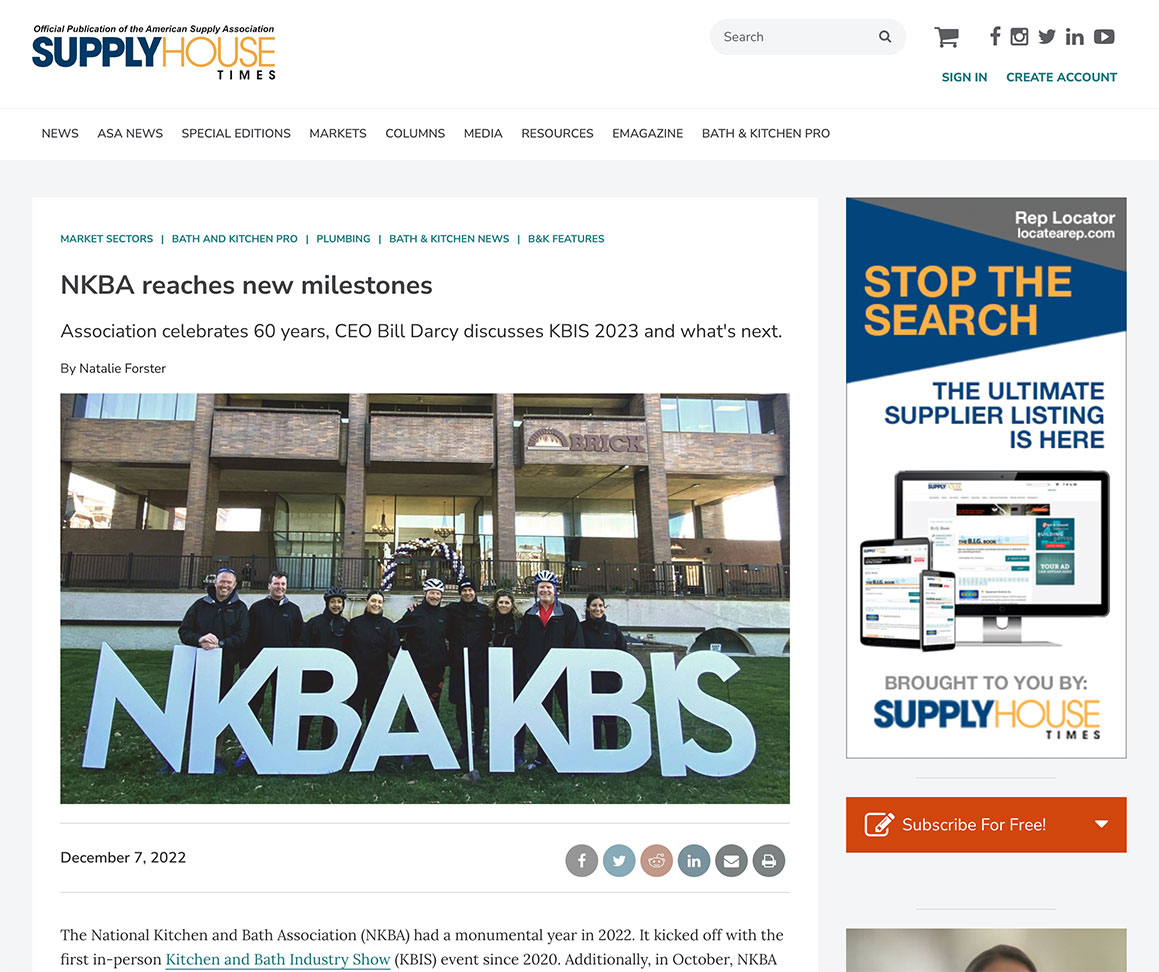This image is a screenshot of the website for the official publication of the American Supply Association, called "Supply House Times." The publication's name is prominently displayed in the top left corner. To the right of this title, there is a search bar and a shopping cart icon, followed by icons for social media platforms: Facebook, Instagram, Twitter, YouTube, and an unfamiliar one. Below these icons are links labeled "Sign In" and "Create Account."

The navigation bar stretches across the top of the page, listing categories from left to right: News, ASA News, Special Editions, Markets, Columns, Media Resources, E-Magazine, Bath and Kitchen Pro. The primary story displayed on the left-hand side features multiple clickable links labeled: Market Sectors, Bath and Kitchen Pro, Plumbing, Bath and Kitchen News, B&K Features. The headline for this story reads "The NKBA Reaches New Milestones: Association Celebrates 60 Years; CEO Bill Darcy Discusses KBIS 2023 and What's Next." Below the headline, there is a photo of a group of people standing behind an NKBA/KBIS sign.

On the right side of the page, there's an advertisement for Supply House. Below this ad, there is a red "Subscribe for Free" button. At the very bottom of the screenshot, part of a picture is visible, showing the top of someone's head.